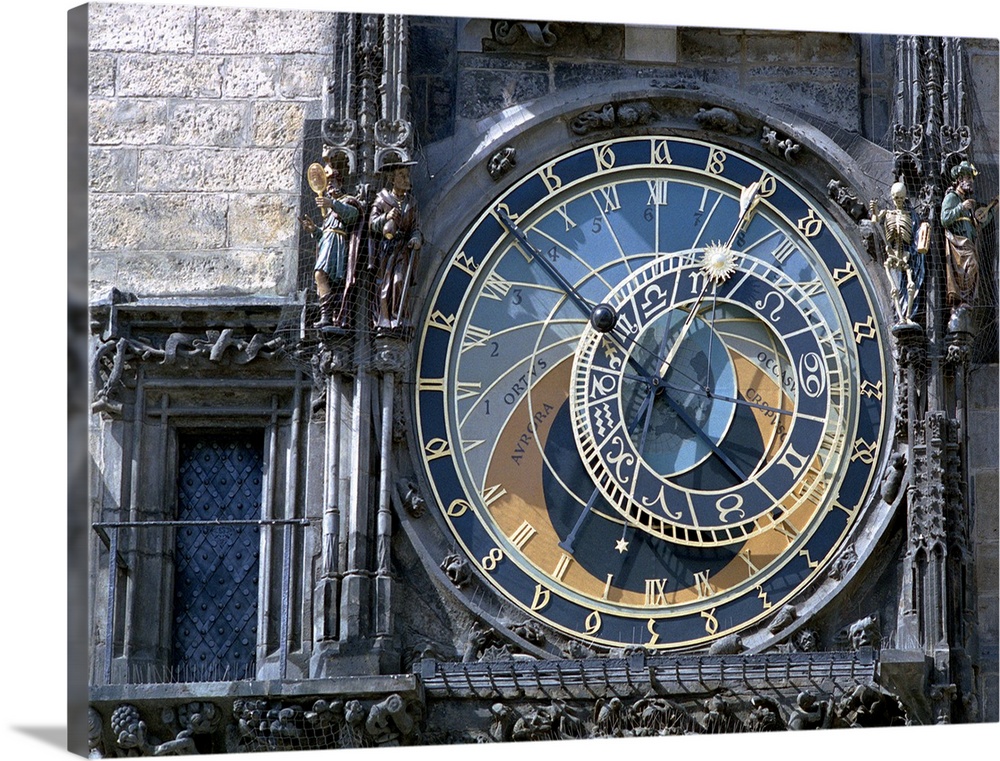A photograph captures an ancient concrete building adorned with an ornate clock that is the centerpiece of the image. The clock face is round and semi-transparent, displaying a mesmerizing gradient of light blues and oranges. Encircling the clock face are gold numerals set against a blue background, indicating hours. Just right of center within the clock face, there's a secondary, smaller circle that features additional symbols and markings. The main clock face is equipped with two black hands, while the smaller inner dial has two goldish hands.

The clock is mounted on a timeworn section of the building, which also features intricate and heavily textured pillars flanking the clock. These pillars exhibit the rugged, aged aesthetic of ancient concrete. Below the clock, an ornamental base with elaborate and detailed designs adds to the historical charm of the structure.

To the left of the clock, a window with a balcony can be seen. The balcony is adorned with spikes designed to deter birds from perching. The overall appearance of the building, including two cement figures positioned on either side of the clock, emphasizes its antiquity and classical architectural style.